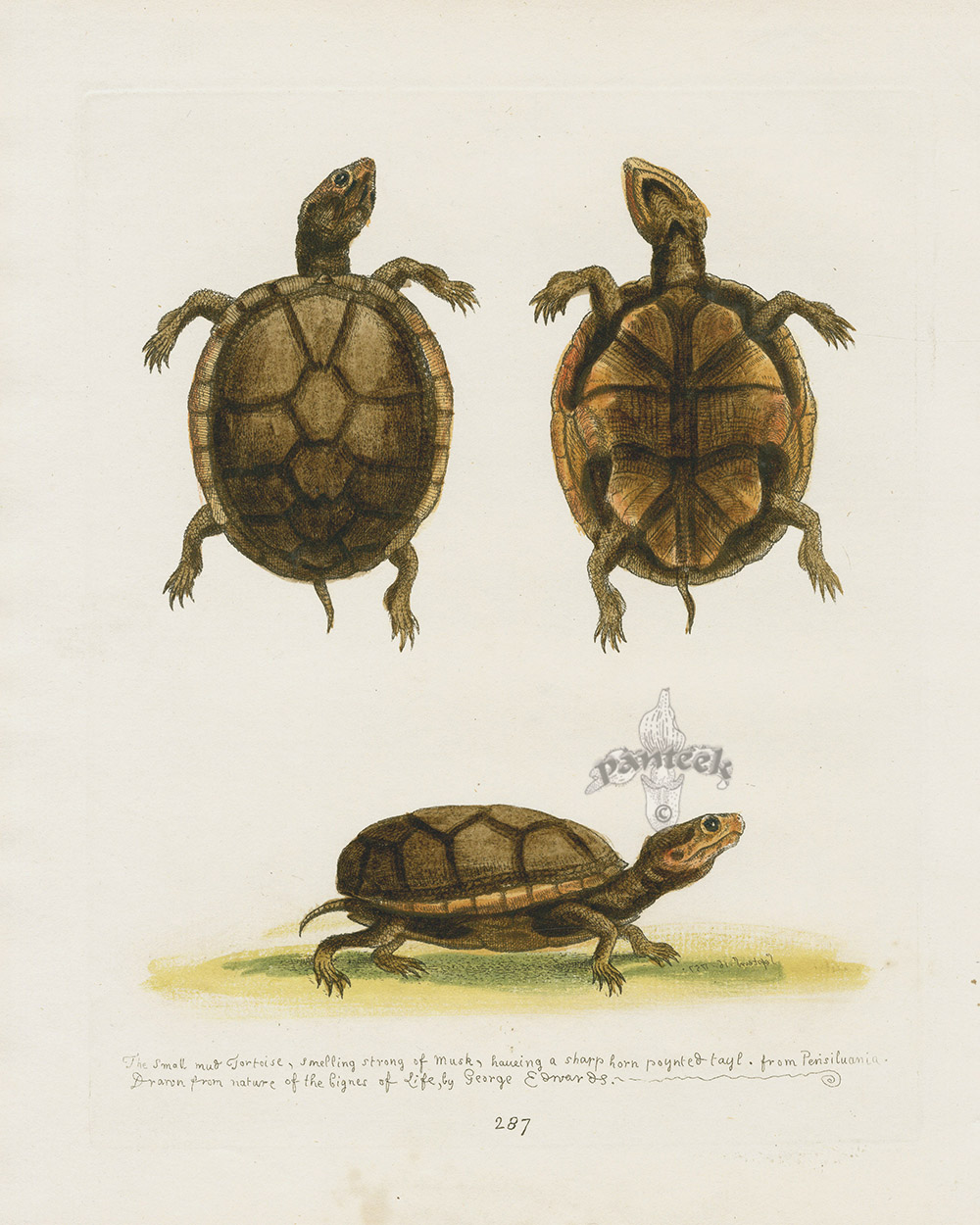This image is an intricate naturalist drawing, crafted with watercolor and colored pencils, and appears to be a historical piece, possibly from the 1850s. The background of the image is a light tan or cream color, adding to its vintage feel. The artwork, attributed to George Edwards, is marked as Page 287 and showcases a small turtle, possibly a common water or mud tortoise from Pennsylvania.

The detailed illustration features three distinct views of the turtle: at the top left, there is the top view highlighting the shell pattern; to the right, the underside view reveals the lower shell anatomy; and at the bottom, the side view shows the turtle standing on the ground, complete with a shadow for depth. The turtle is depicted in shades of brown and gray-green, with lighter brown accents around the edges of the shell and sides of the face.

Handwritten text at the bottom of the image describes the turtle as "The small mud tortoise, smelling strong of musk, having a sharp horn and pointed tail." Additionally, there is a logo or watermark reading "Pantique," possibly over an orchid or exotic flower, which appears to be done in pencil.

All these elements combine to provide a comprehensive and detailed representation of the turtle from multiple perspectives.